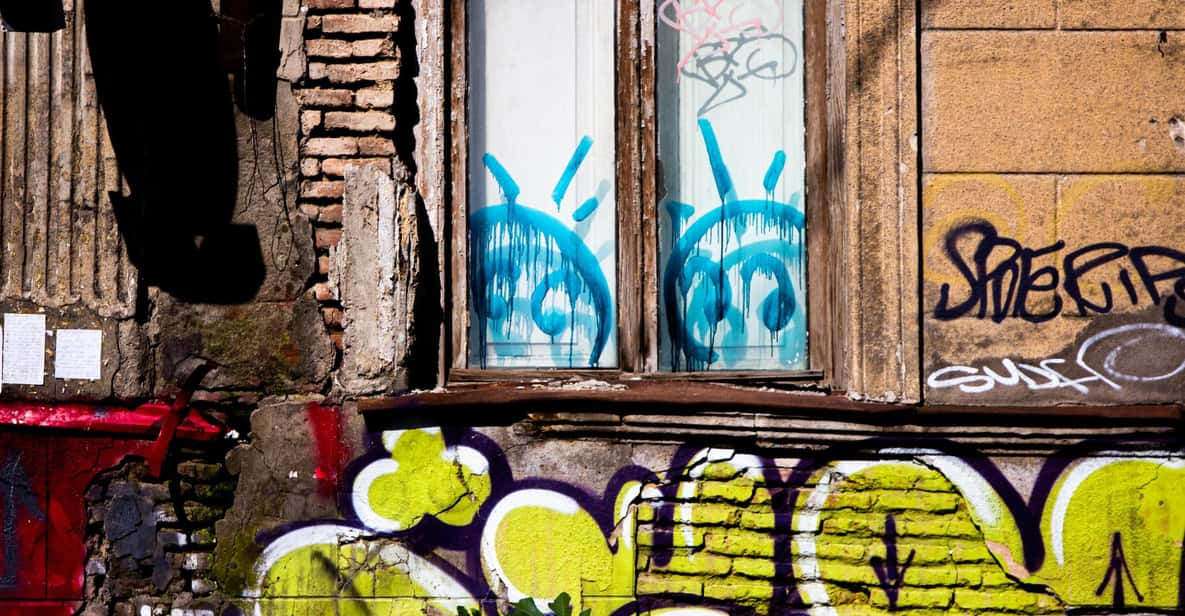The photo captures a side wall of an old, possibly abandoned building that has seen better days. The structure appears weathered, with parts of the masonry broken off, exposing bricks and cracked stone underneath. The facade is a patchwork of colors, with a dominant presence of graffiti that covers much of its surface, including the boarded-up windows. There are two thin windows, one on the left and one on the right, each featuring painted figures resembling simplified faces or alien-like creatures. These faces are light blue circles with three lines atop them, somewhat evocative of sun rays or head antennae. Surrounding these windows are various graffiti writings in multiple colors, including black, yellow, neon green, and red. The lower part of the wall is adorned with large, bubbly-style graffiti letters, primarily painted in yellow with outlines in white and black, creating a striking contrast. Although some of the black and white graffiti text is somewhat decipherable, the overall impression is one of a vibrant, if chaotic, urban art scene.